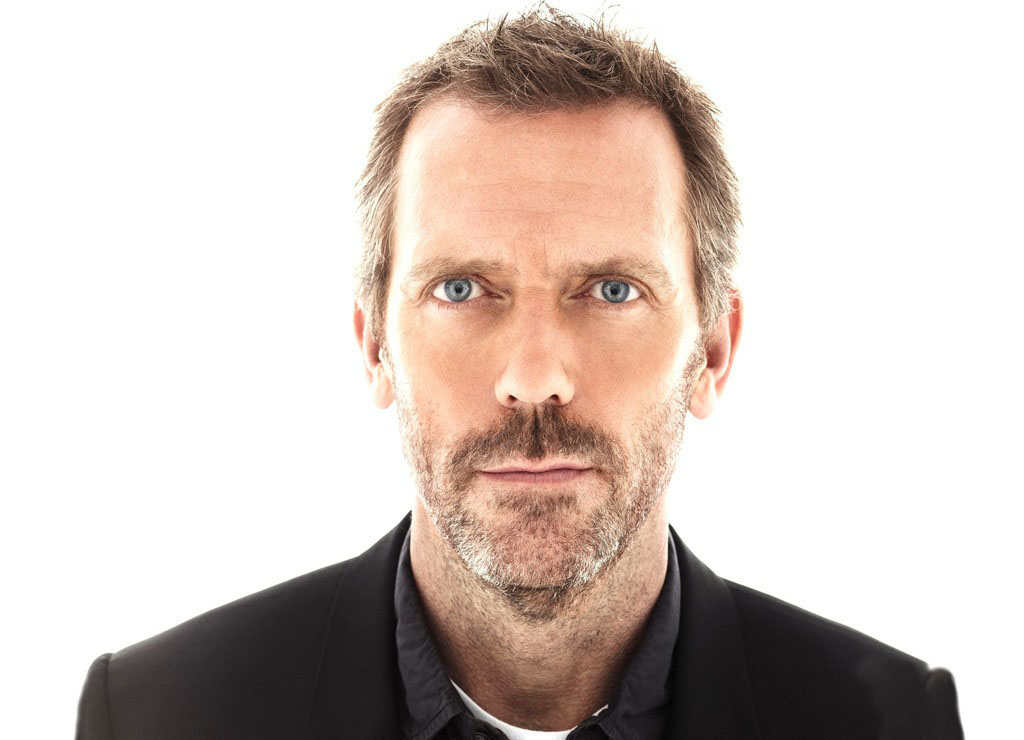Here we have an image of the actor known for his role in the show House M.D. He has short brown hair with a hint of gray and some hair slightly sticking up in the middle. The actor is staring directly into the camera with his piercing blue eyes, wearing a very serious expression. His facial hair consists of a scruffy goatee and beard, with additional scruff visible on his neck, indicating he hasn't shaved cleanly. 

He is dressed in a black suit jacket paired with a black collared shirt, and underneath that, there's a glimpse of a white t-shirt. The picture mainly captures the area above his chest and shoulders, set against a simple white background. The overall look is one of a slightly unkempt but serious man, reminiscent of his character's demeanor in the show.